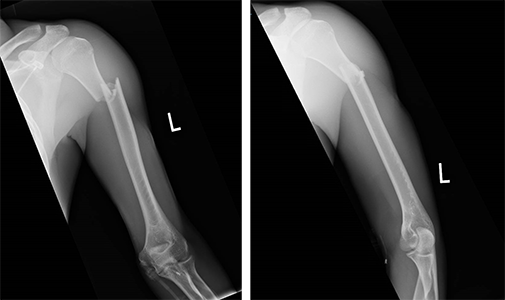This image contains two x-rays of a left arm, set against a completely black background. Both x-rays are marked with the letter "L," indicating they are of the left arm. The x-ray on the left shows a broken arm bone located just below the shoulder, with the fracture completely severing the bone. The right x-ray depicts the same arm after medical intervention, illustrating the bone in a healing or healed state, having been correctly set back in place. You can still see the outline of the previous fracture site. The left x-ray is darker, while the right x-ray appears fuzzier but shows more anatomical detail, including some muscle outlines.